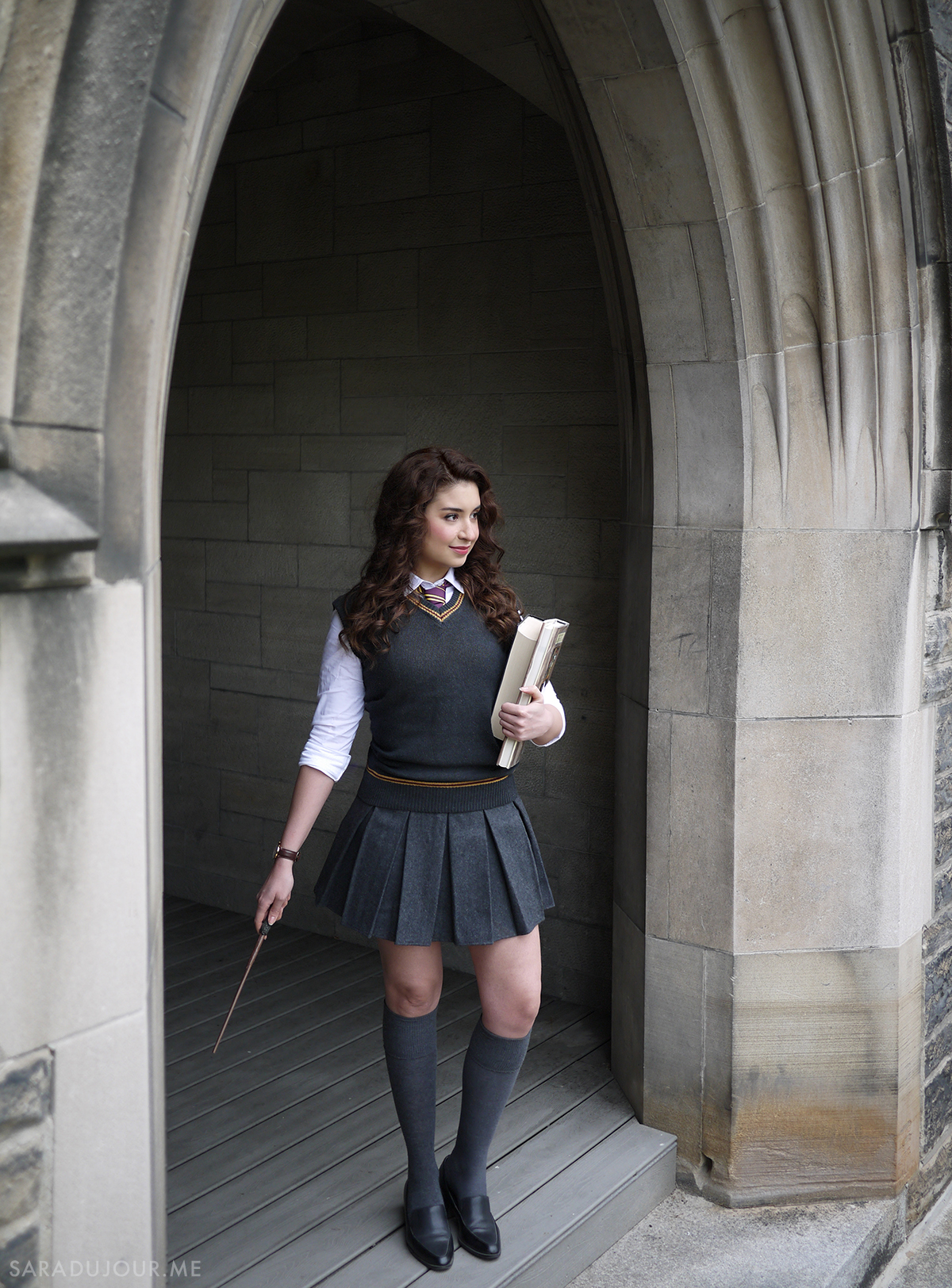This is a detailed photograph of a young woman cosplaying as a character from Harry Potter, standing in an arched doorway of a stone building. The floor of the building is made of gray wooden planks. She exudes a scholarly aura with her long, curly brunette hair flowing down to her shoulders. She is dressed meticulously, wearing a white button-down blouse with a burgundy tie that has a yellow stripe. Over the blouse, she dons a gray vest embellished with a yellow strip at the bottom and a V-neck. Her outfit is completed with a short gray pleated mini skirt, knee-high gray socks, and black slip-on shoes. On her right wrist, she wears a black wristwatch.

In her right hand, she holds a wand pointed downward, while her left hand clutches two textbooks against her chest. She faces to the right, exuding a slight smile. The backdrop of a light gray stone archway, comprised of various-sized rectangular bricks, adds a historical touch to the image, with shadows in the background creating depth. Notably, at the bottom left of the photograph, the white text "sarahdujour.me" is inscribed, suggesting the origin or credit for the image.